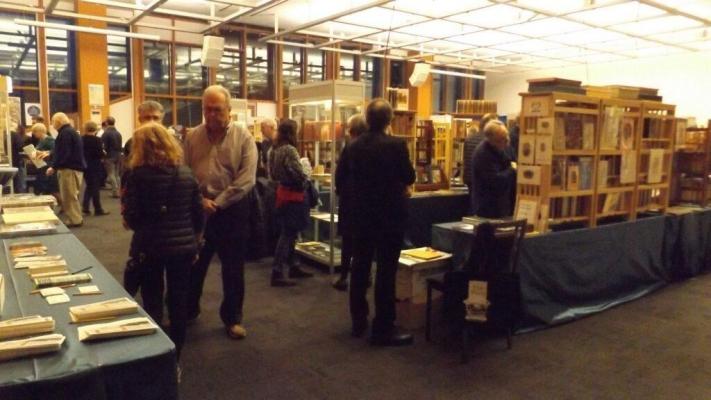This is an older color photograph depicting an indoor book fair or literary exhibition, likely from the 1990s or early 2000s, as indicated by the slightly yellowed hue and lower image quality. The setting is a large, luminous hall, possibly a library or a bookstore, with a grid of ceiling lights casting a bright, fluorescent glow. Along the hall, numerous long tables are covered with black or blue tablecloths, each adorned with pamphlets, pencils, brochures, and several display stands showcasing books, artwork, and prints encased in protective sleeves.

An eclectic group of 15 to 20 mostly middle-aged to older Caucasian attendees mill about, examining the items on display, engaging in conversations, and interacting with vendors. Key figures include a lady with blonde hair dressed in a black jacket and pants conversing with a man in glasses, a gray shirt, black pants, and brown shoes, while a man in a black suit stands nearby with his back to the camera. Another individual, dressed in a black jacket and noticeably balding, is intently examining a bookshelf labeled "2," holding various books or artworks.

In the backdrop, large windows with brown paneling allow natural light to seep in, further illuminating the scene. The floor is covered in industrial carpeting, grounding the viewers in this bustling yet intimate venue, highlighted by a mix of modern and nostalgic elements.